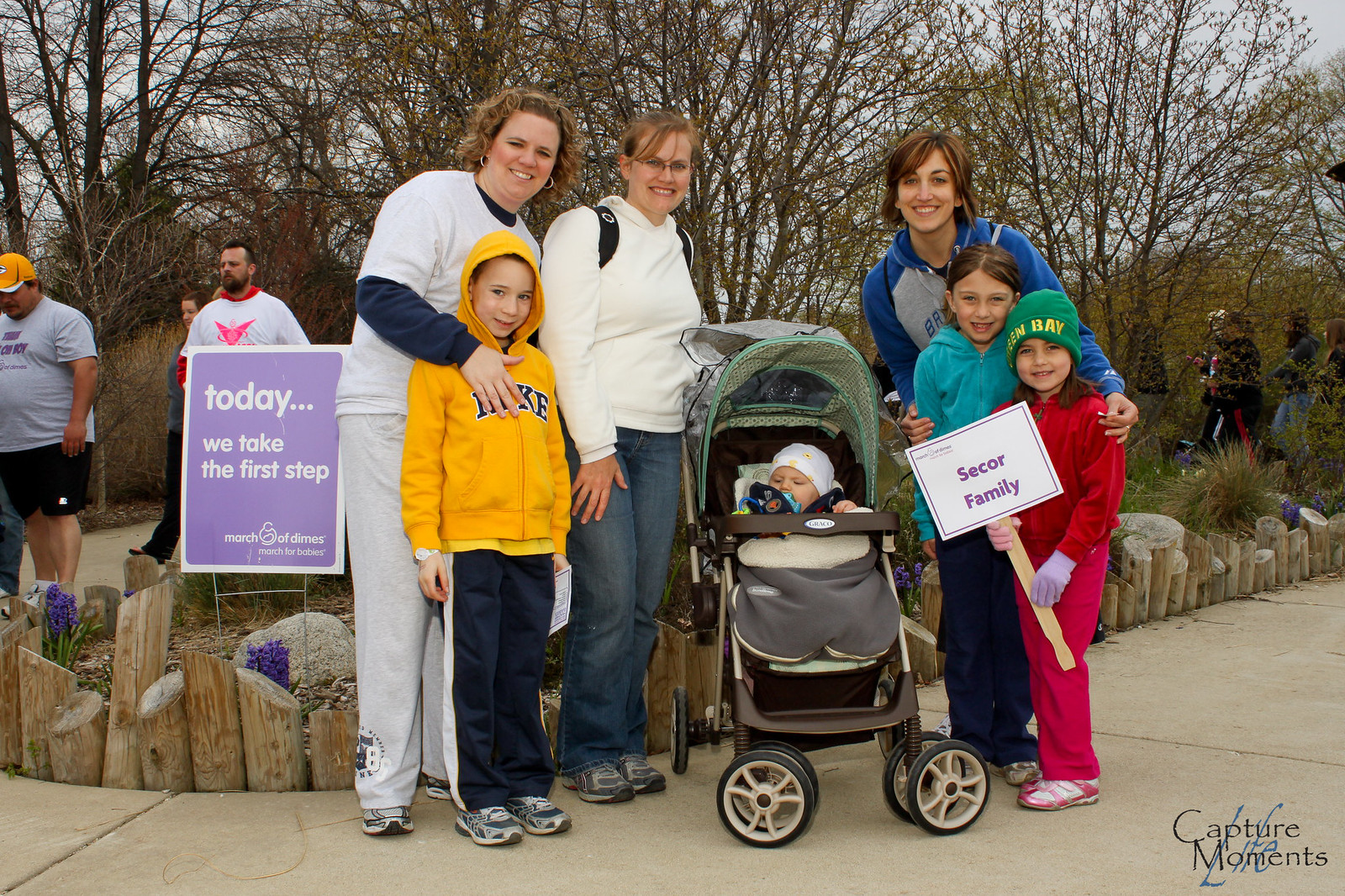A group of seven people is posing for a photograph on a tree-lined sidewalk, participating in a March of Dimes event. To the left, a curly-haired woman in a blue long-sleeved shirt layered under a white short-sleeved shirt and gray sweatpants has her left arm around a young boy standing in front of her. The boy is sporting a yellow Nike sweatshirt with the hood up, blue pants featuring a white stripe, and tennis shoes. Next to them is a woman with light brown hair, wearing a white hoodie, blue jeans, gray shoes, and glasses, carrying a backpack over her shoulders. 

To the right of this woman is a baby in a green-topped stroller, wearing a white hat with a pacifier in its mouth and covered with a gray blanket. Three additional individuals stand beside the stroller. Closest to the stroller is a woman with short brown hair, smiling at the camera and dressed in a blue and gray hoodie. In front of her stands a younger girl with long brown hair parted down the middle, wearing a turquoise hoodie and blue pants. In front of this girl is a little girl in a red jacket and red pants, sporting a green hat with yellow letters, holding a white sign with purple letters reading "SECOR FAMILY."

Behind the group, there are trees and a visible pathway where other participants of the event can be seen walking. A purple sign on the left side of the photo reads "Today we take the first step, March of Dimes, March for Babies." Additionally, the bottom right-hand corner of the image features the text "Capture Moments."